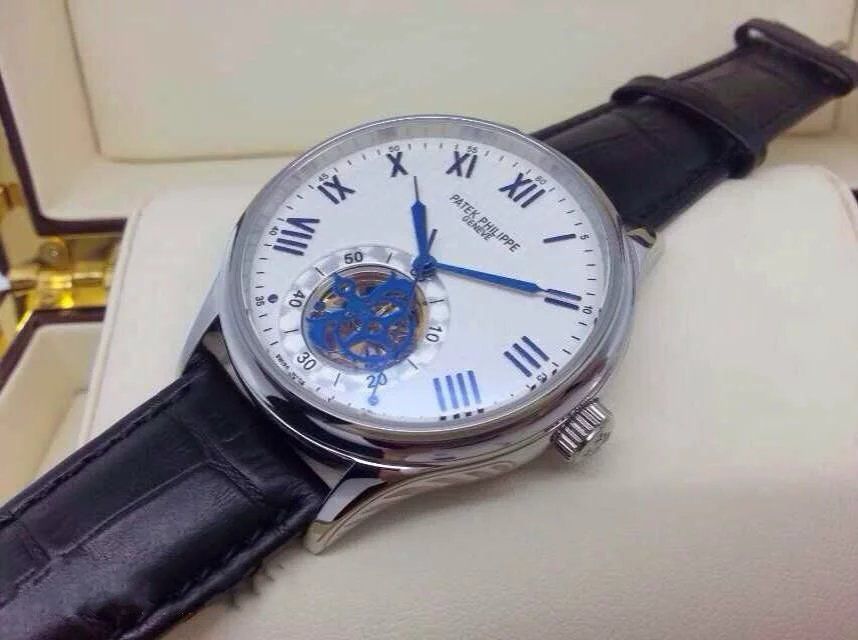This detailed photograph captures an elegant Patek Philippe Geneve men's analog wristwatch prominently displayed in its open white display box. The watch exudes sophistication with its mix of silver, white, black, and navy blue colors. The bezel is clear crystal, allowing an unobstructed view of the white face adorned with blue Roman numerals marking the hours. The watch's hands and the small dial at the bottom center, which likely tracks seconds, are in a striking cobalt blue. Enhancing the watch's allure is an opening that reveals blue gears and additional markings for 10, 20, 30, 40, and 50 seconds. The watch sports a sleek black leather band, contrasting elegantly with the light background. The silver crown for time adjustments is situated on the right side. The case's lid is slightly visible in the background, suggesting the watch's readiness for display or focused admiration. The intricate details and high-quality craftsmanship make this timepiece an emblem of luxury and precision.